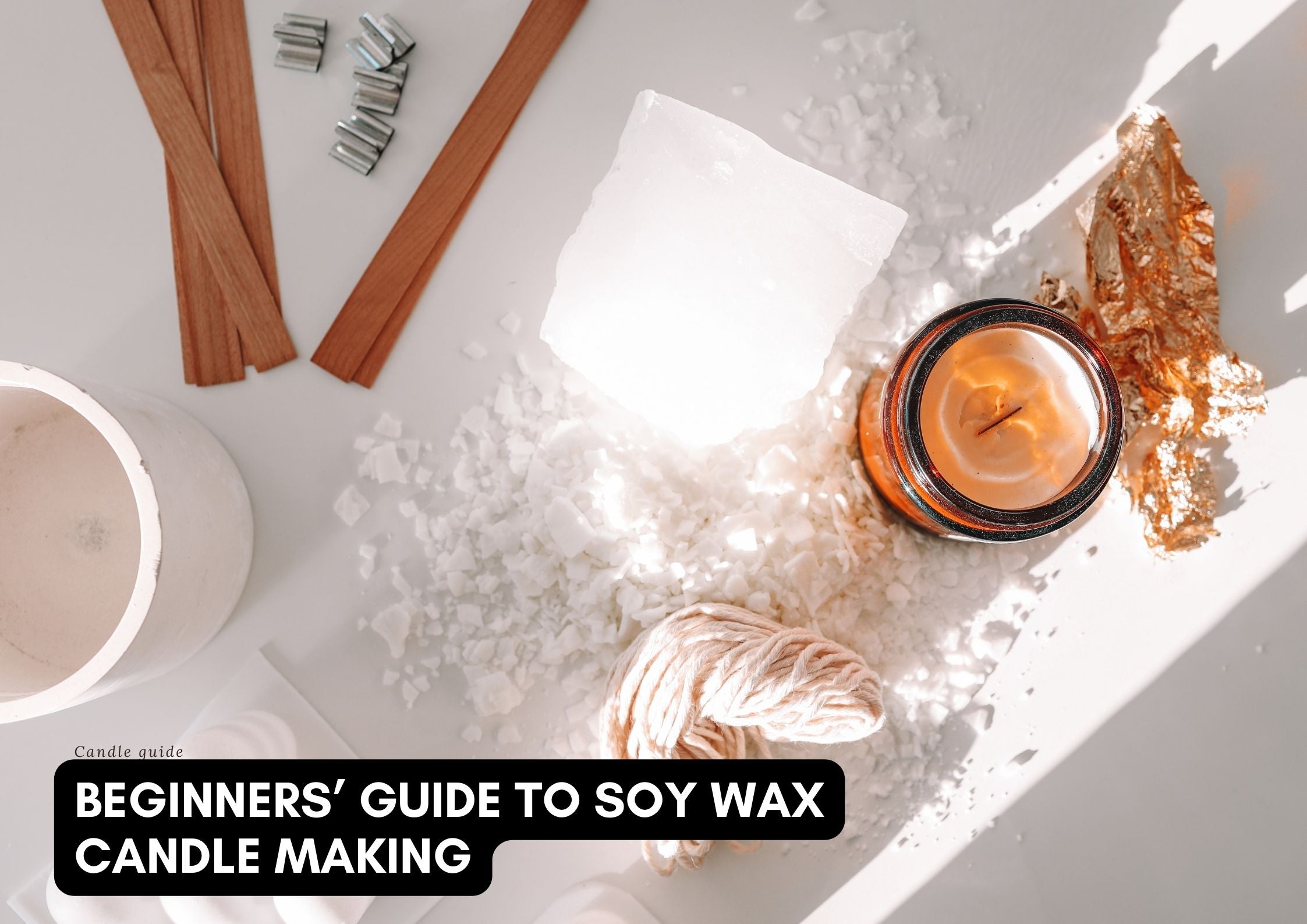The image showcases a meticulously arranged collection of items on a pristine white surface, all associated with candle making. In the bottom left corner, a black-bordered section with white text prominently reads, "Beginner's Guide to Soy Wax Candle Making," with "Candle Guide" above it in a delicate black serif font. To the left, a rounded white jar stands, while above it and slightly to the right lie several thin, reddish-brown wooden shims. Nestled between these shims are four small, silvery T-shaped molds. Below these, a pile of crumbly white material surrounds a large, translucent white block, suggesting raw soy wax. Moving to the right, a reddish-brown glass jar filled with a candle-like white substance sits adjacent to a glittering pile of gold foil. Near the bottom of the frame, a neatly coiled white ball of string, likely a candle wick, is visible. The detailed arrangement and varied elements provide a comprehensive view into the tools and materials essential for soy wax candle making.